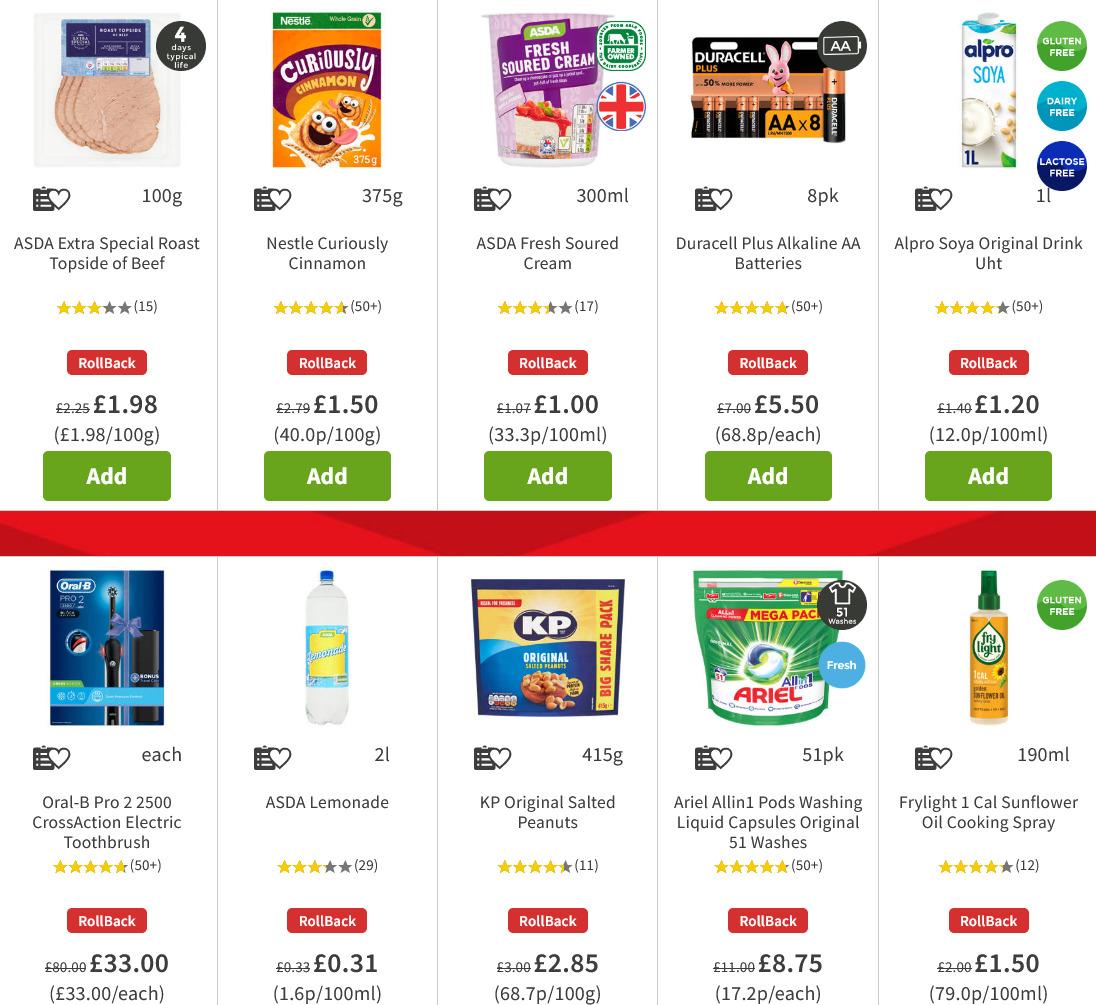Here's a polished and detailed caption for the image depicting products on a shopping site:

---

This screenshot from a shopping site showcases ten products arranged in a five-by-two grid. Each product tile includes an image, star rating, "Roll Back" label in a red box, price, and an 'Add' button in green.

Top Row, Left to Right:

1. **ASDA Extra Special Roast Topside of Beef**: Featuring a near-perfect star rating alongside a "Roll Back" label. Priced at £1.98 per pound with a convenient green "Add" button for easy purchase.

2. **Nestlé Curiously Cinnamon Cereal**: Boasts an almost five-star rating, indicated by yellow stars. Marked with a "Roll Back" label and priced at £1.50 per pound. Includes a green "Add" button.

3. **ASDA Fresh Sour Cream**: Displayed with a solid star rating, a "Roll Back" label, and a promotional price of £1.00. The green "Add" button makes adding to your cart seamless.

4. **Duracell Plus Alkaline AA Batteries**: Highlighted with a five-star rating. The "Roll Back" label indicates a reduced price of £5.50. Features a green "Add" button.

5. **Alpro Soya Original UHT Drink**: Presented with star rating and "Roll Back" label. It is priced at £1.20. Information bubbles indicate it's gluten-free, dairy-free, and lactose-free. The green "Add" button is also present.

Bottom Row, Left to Right:

1. **Oral-B Pro CrossAction Electric Toothbrush**: Priced at £33.00.

2. **ASDA Lemonade**: Showcases star rating and "Roll Back" label. Priced at £0.31 per bottle.

3. **KP Original Salted Peanuts**: Accompanied by a star rating and "Roll Back" label. Available at £0.85 per pack.

4. **Ariel All-in-1 PODS Washing Capsules (Original, 51 Washes)**: Features star rating and "Roll Back" label, priced at £8.75.

5. **Frylight 1 Cal Sunflower Oil Cooking Spray**: With star rating and "Roll Back" label. It is priced at £1.50.

Each product tile is designed to give clear, detailed information, making it easy for customers to evaluate and add products to their shopping carts.